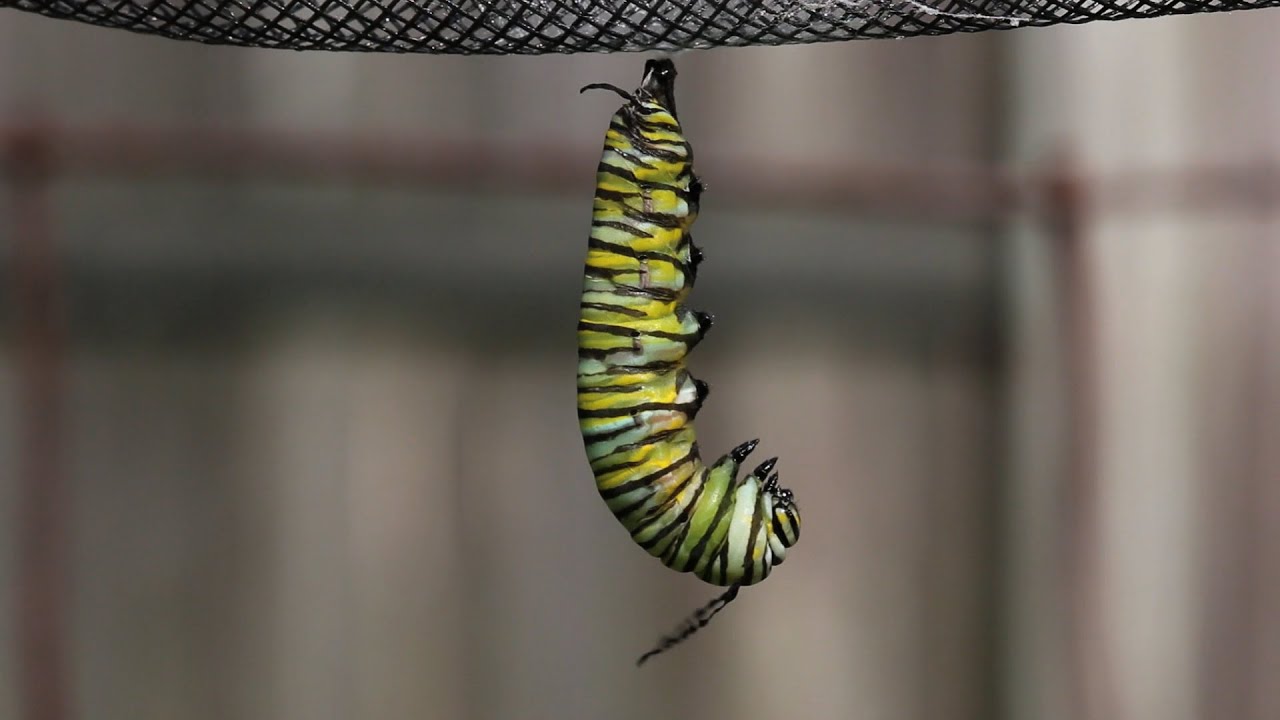This detailed photograph features a colorful caterpillar, likely a monarch butterfly caterpillar, hanging upside down from a black mesh or netting. The caterpillar, adorned with vivid bands of light green, pea green, white, black, and yellow, is attached by its back end, with its head and tiny appendages dangling downward. This setup suggests that the caterpillar is preparing to form a chrysalis for pupation. The background of the image is heavily blurred in shades of tan and gray, possibly hinting at an indoor environment such as a breeding tank or cage, although the exact setting remains indistinct. No additional labeling or wording is present in the photograph.